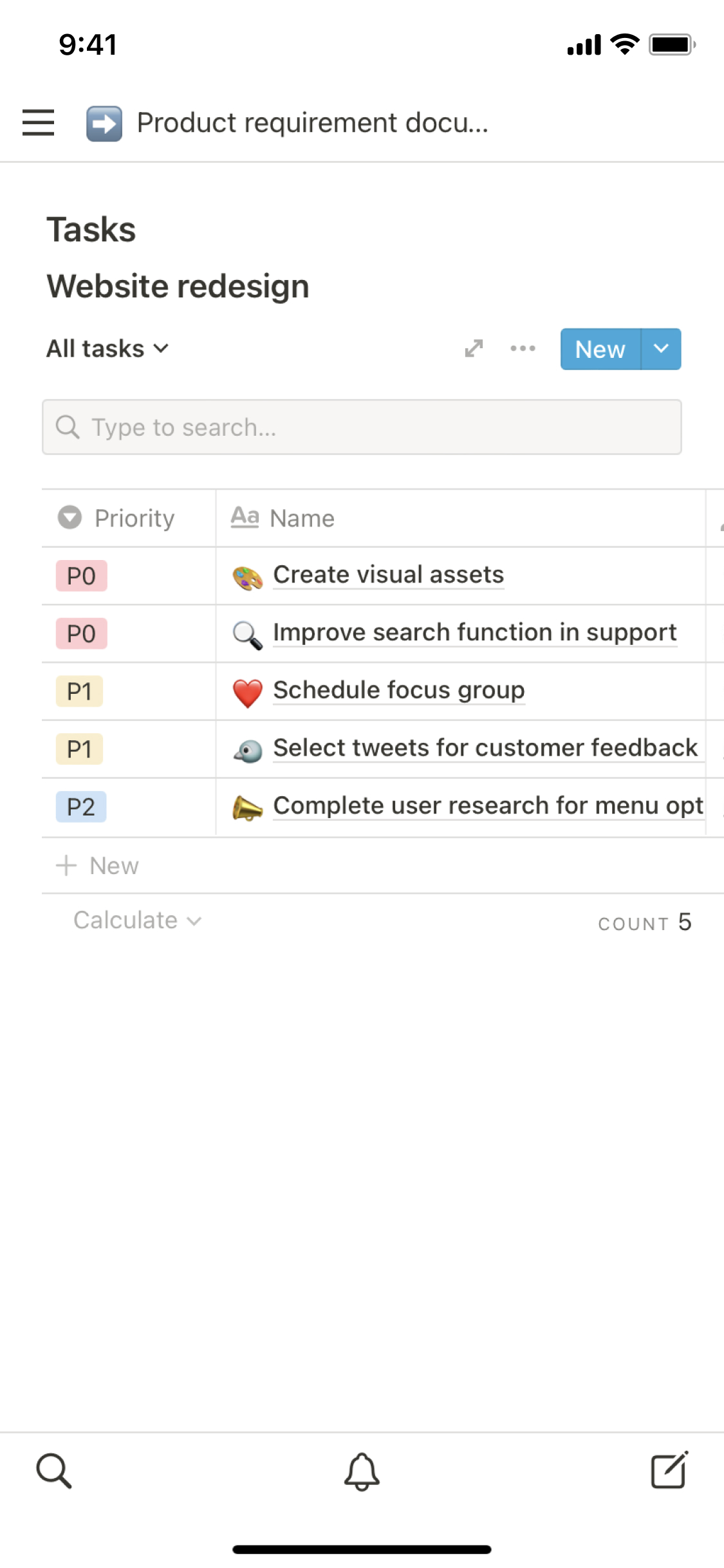The image features a task management interface with various elements. At the top left corner, bold black text reads "941". To the top right, there are four fully charged battery icons labeled "GE". Directly below this is a set of three black menu bars on the left and a metallic right-pointing arrow on the right. 

The section immediately beneath this reads "Product with Requirement Docu..." in black text. Below it, "Tasks" is written in black text, and then "Website Redesign" is prominently displayed in bold black text. Another line in bold black text reads "All Tasks" followed by a right-pointing arrow below this text.

Further down, there is an arrow stretching up to the right and down to the left, accompanied by three additional arrows. The words "New" are hyperlinked in bold red and blue text, along with a button labeled "New" to the right of it.

Below this, there is an empty search bar in grey with the placeholder text "Type to search..." in grey default text. Underneath the search bar, there is a list of priorities labeled as "Priority," with specific items tagged as P0, P0, P1, P1, and P2. The priority colors are as follows: P0 in orange, P0 in red, P1 in orange, and P2 in blue. Immediately to the right of the two P0 labels, issues are described as "Create Visual Assets" and "Improve Search Function."